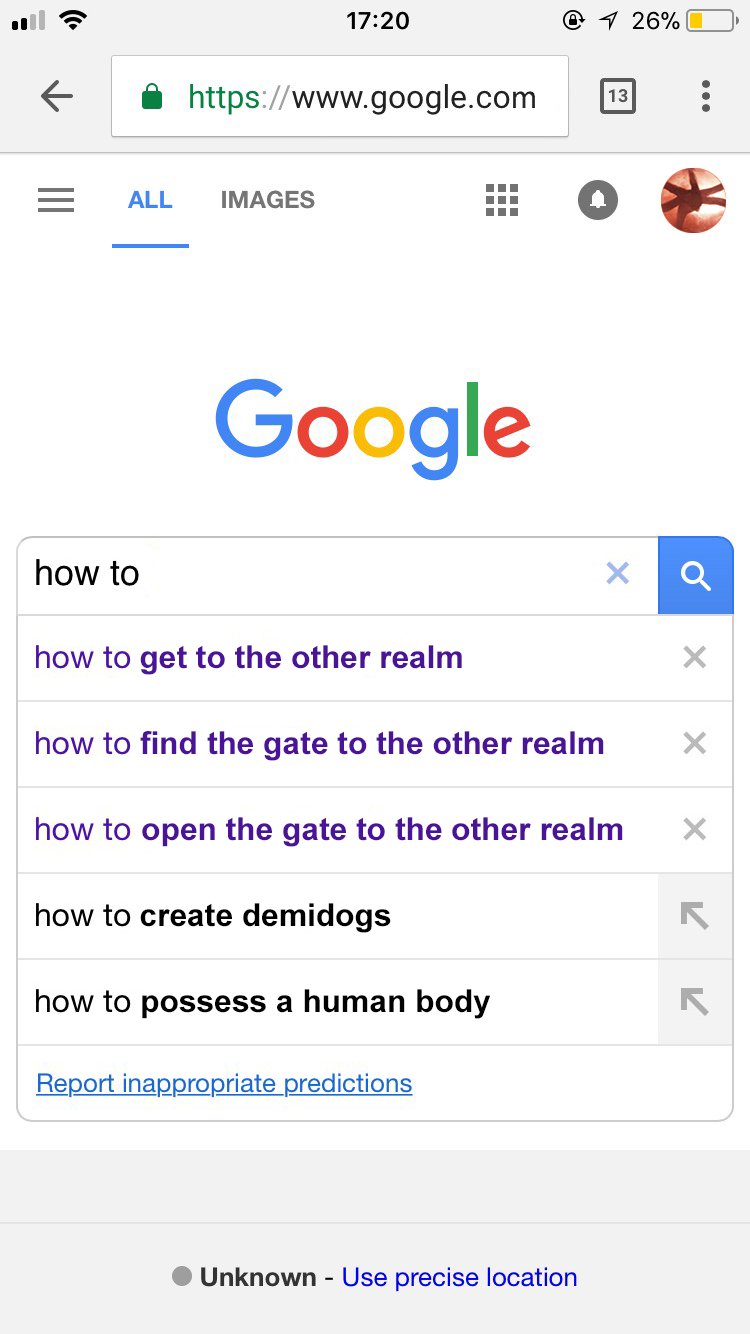The image depicts a computer screen capturing a Google search session. At the very top of the screen, there are multiple browser tabs open alongside standard interface elements including the time, battery status, and WiFi connectivity. Below this header section, a familiar Google homepage is visible, with the iconic "Google" logo prominently displayed in large font. In the search bar, partially visible, are the words "how to".

In the main search results area, a circle with an image that resembles a spider is present on the right side. The search query includes several unusual and specific queries: "How to get to the other realm," "How to find the gate to the other realm," "How to open the gate to the other realm," "How to create demidogs," and "How to possess a human body." 

Finally, at the very bottom of the screen, there is text indicating a prompt for "unknown use precise location" and an option to "report inappropriate predictions." This detailed search query results in a peculiar and slightly eerie context, suggesting a user delving into supernatural or fantasy themes.